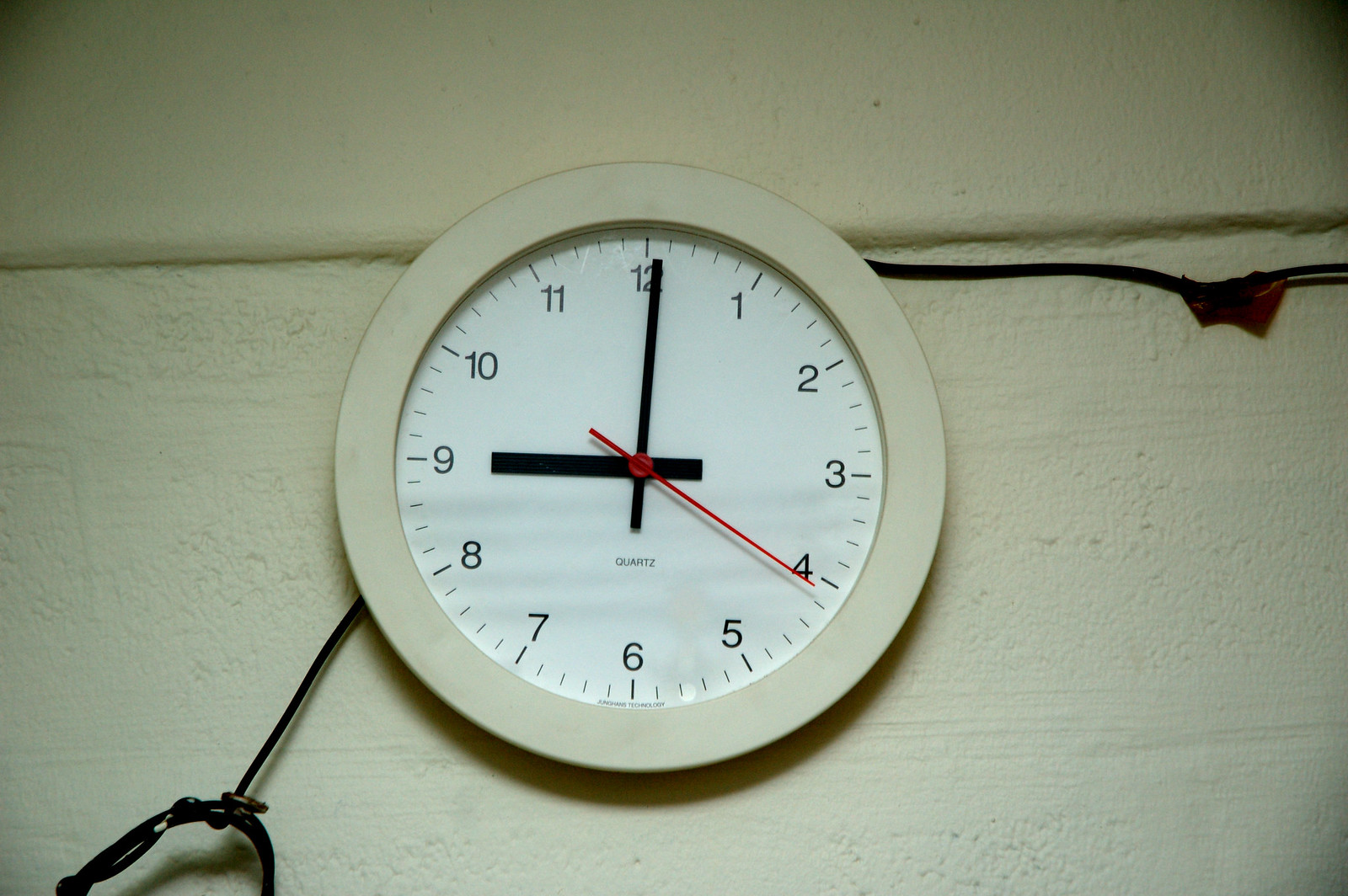This close-up photograph depicts a simple, round clock mounted on a rough-textured, white-painted wall. The clock case is a slightly dirty cream color, potentially made of plastic, with a white face. Black numbers mark 1 through 12 with lines above each and four smaller lines between each number to denote minutes. The time is precisely 9 o'clock and 21 seconds, indicated by plain black hour and minute hands, and a red second hand. The word "quartz" is inscribed in black letters beneath the hands. The clock is accompanied by visible black electrical wiring, with a cable running down vertically and then across horizontally, some of which is wrapped in colored electrical tape.